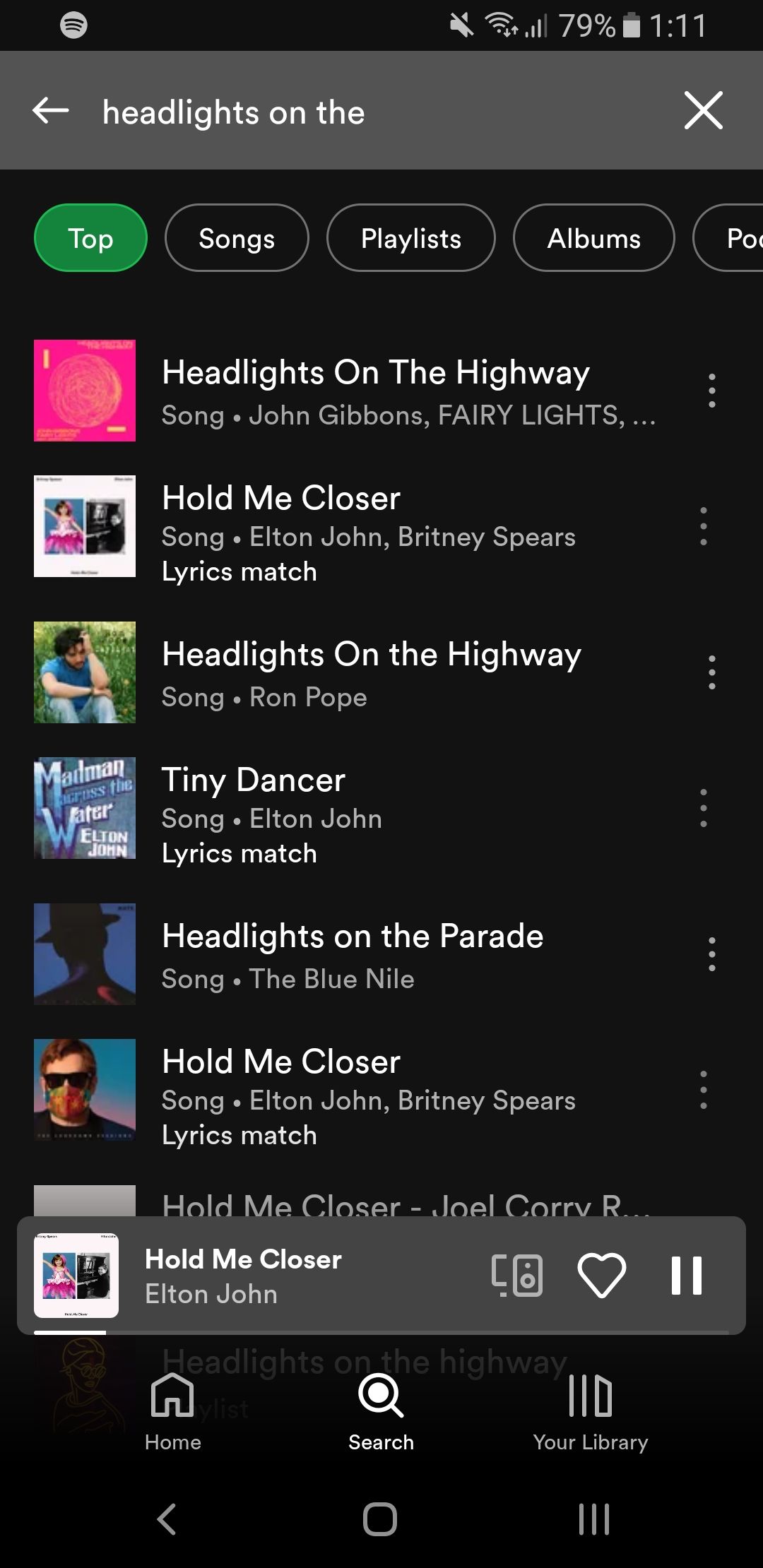This is a detailed descriptive caption for the image provided:

---

This image is a screenshot taken from a mobile phone displaying the Spotify app with a black background. At the very top of the screen, there is a black status bar containing information about the phone. On the left side of this bar, the Spotify logo is visible, which consists of a white circle with three curving black lines inside it. To the right of the logo, there are several icons indicating the phone’s current status: a microphone icon with a slash through it, a WiFi icon, a mobile signal strength icon, and a battery icon showing the battery level at 79%. The current time displayed is 1:11.

Below this status bar, there's a gray search bar where users can search within Spotify. The text "headlights" is typed into this field. To the left of the search bar, there is a white arrow pointing left, which functions as a back button, and to the right is an 'X' icon that allows users to clear the search field.

Underneath the search bar, there is a row of selectable filter buttons labeled "Top songs," "Playlists," and "Albums." The "Top" button is highlighted in red, indicating it has been selected. As a result, the screen displays a list of top songs containing the word "HEADLIGHTS" in their titles. The top song in this list is "HEADLIGHTS ON THE HIGHWAY" by John Gibbons.

---

This descriptive caption provides a thorough depiction of the screenshot, detailing the layout and specific elements visible within the Spotify app.